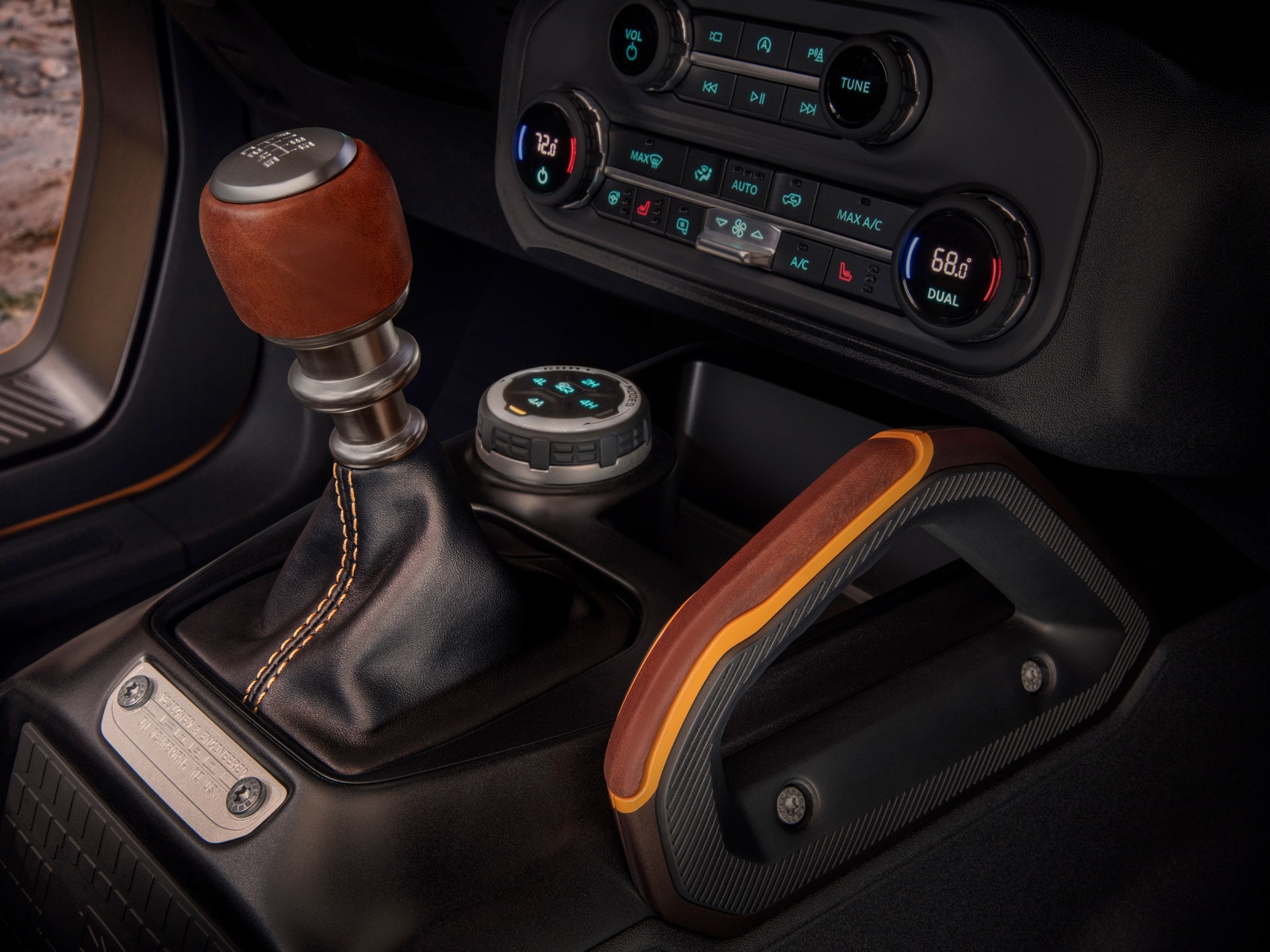This close-up photograph captures the intricate details of a sporty car's center console, showcasing a blend of luxury and functionality. The focus is on a distinctive manual gear shift, featuring a unique design resembling a large screw. The shift knob is crafted from a brownish wood material with a brushed silver top displaying the gear positions. The metal shaft of the gear shift descends into a black leather-covered base, integrating seamlessly with the modern aesthetic of the console. Surrounding the gear shift are typical car functions, including a round, multifunctional control knob likely for the radio, push-button controls, and illuminated climate controls. The left seat warmer is set at 72 degrees while the right is at 68 degrees. The interior, highlighted by black and metal elements, underlines the car's sporty and sophisticated design. The detailed, hyper-realistic nature of this image suggests it might be a stylized art piece or a computer-generated illustration, adding a layer of modernity to the vehicle's interior depiction.